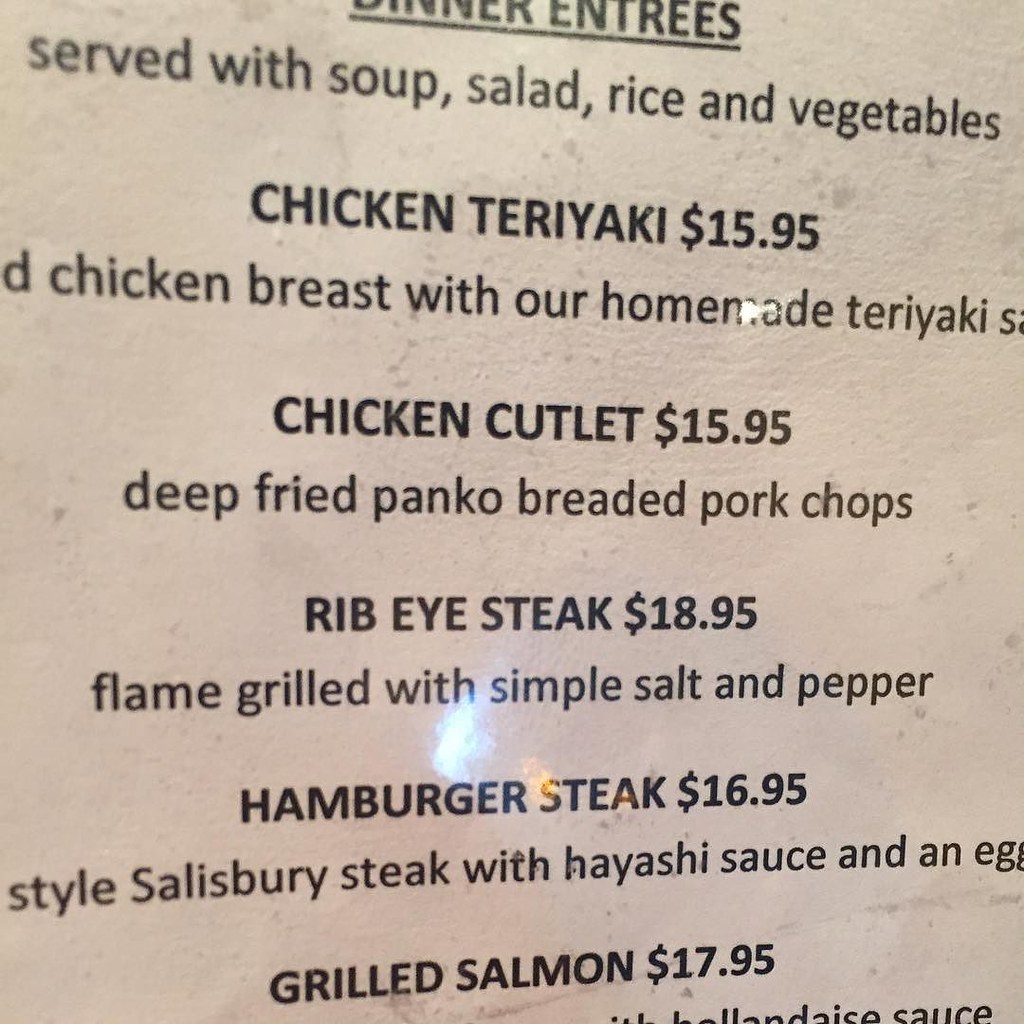The image is a close-up of a restaurant menu. The top part of the menu is partially cut off, but it likely reads "Dinner Entrées" in black text, underlined. Below that, in black text, it states that the dishes are "Served with soup, salad, rice, and vegetables." 

The listed entrees and their descriptions are as follows:

- **Chicken Teriyaki - $15.95**  
  Chicken breast with homemade teriyaki sauce (the remaining description is cut off).

- **Chicken Cutlet - $15.95**  
  Deep-fried, panko-breaded pork chops (ends mid-sentence, and additional text is not visible).

- **Ribeye Steak - $18.95**  
  Flame-grilled with simple salt and pepper.

- **Hamburger Steak - $16.95**  
  Styled like Salisbury steak with hayashi sauce and an egg.

- **Grilled Salmon - $17.95**  
  (The description is not visible as the text cuts off at this point).

The menu text is presented primarily in black, with the names of the dishes in bold for emphasis.